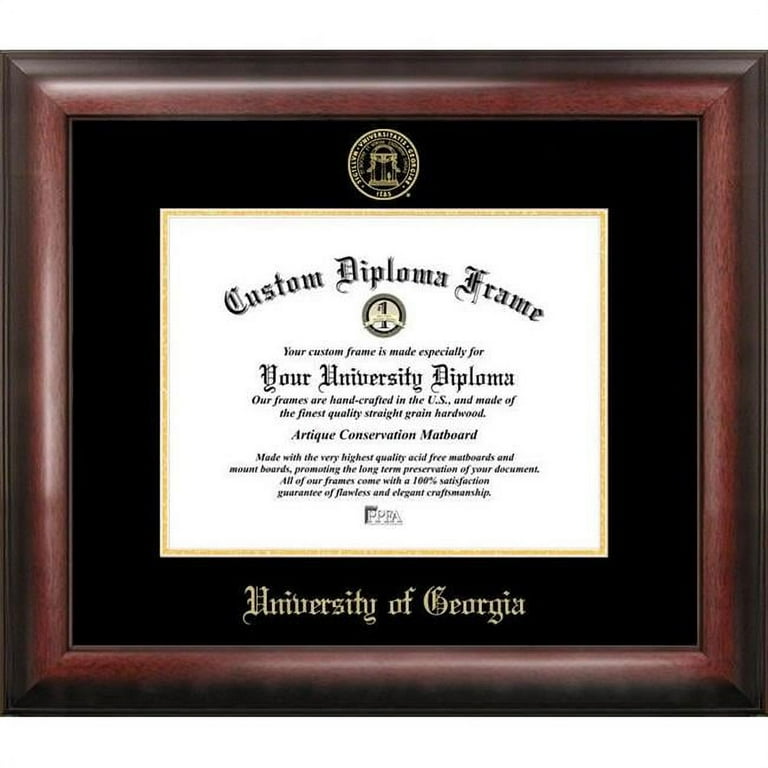This image showcases an elegantly framed diploma, designed as a sample display. The frame, made of dark wood with a hint of reddish tone—possibly cherry or mahogany—features beveled edges and precise miter joints at the corners. Centered within the frame is a black mat with gold trim, enhancing the overall aesthetic. At the top of the mat, there is a college logo embossed in gold. The sample diploma inside the frame prominently reads "Custom Diploma Frame," followed by a description stating that the frame is handcrafted in the US from the finest quality straight grain hardwood, designed specifically for university diplomas. It also mentions the use of the highest quality acid-free mat boards and mount boards to promote long-term document preservation. Additionally, the frame craftsmanship is guaranteed to be flawless and elegant. At the bottom of the mat, in gold text, it reads "University of Georgia," beneath which it states, "Go Dawgs!" emphasizing its affiliation. This setup is positioned as an advertisement, illustrating exactly where a diploma could be showcased after graduation.